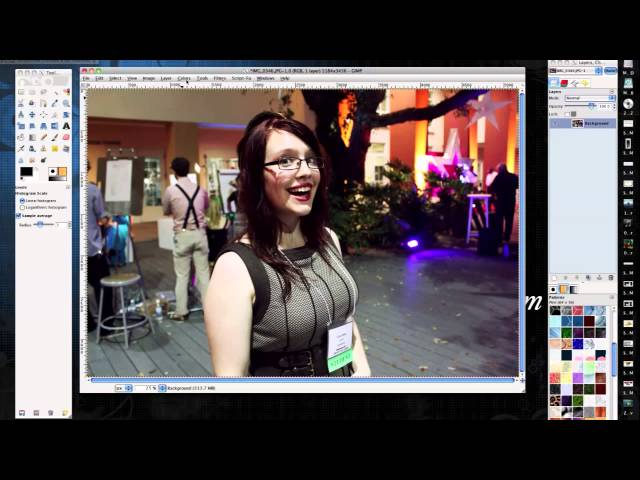This screenshot from a computer screen appears to show an interface for photo manipulation, with numerous icons and tools suggesting functions similar to those found in design software, although it's not Photoshop. The interface is framed by thick black borders at the top and bottom. On the left and right sides, there are vertical white rectangles containing various tools, drawing icons, and color options. The center of the screen features a photo of a woman smiling broadly. She has light skin, dark brown hair that might have a purple tint, and small black-rimmed glasses. She wears a black and white sleeveless top and dark lipstick, with a name badge hanging around her neck. The name badge is white, black, and mint green, hinting she might be at an event, possibly an art gallery. The background suggests an indoor setting with a large tree, gray wooden flooring, and several people, including a man in khaki pants and suspenders. Decorative elements like stars and lights hang from the ceiling, adding to the ambiance.